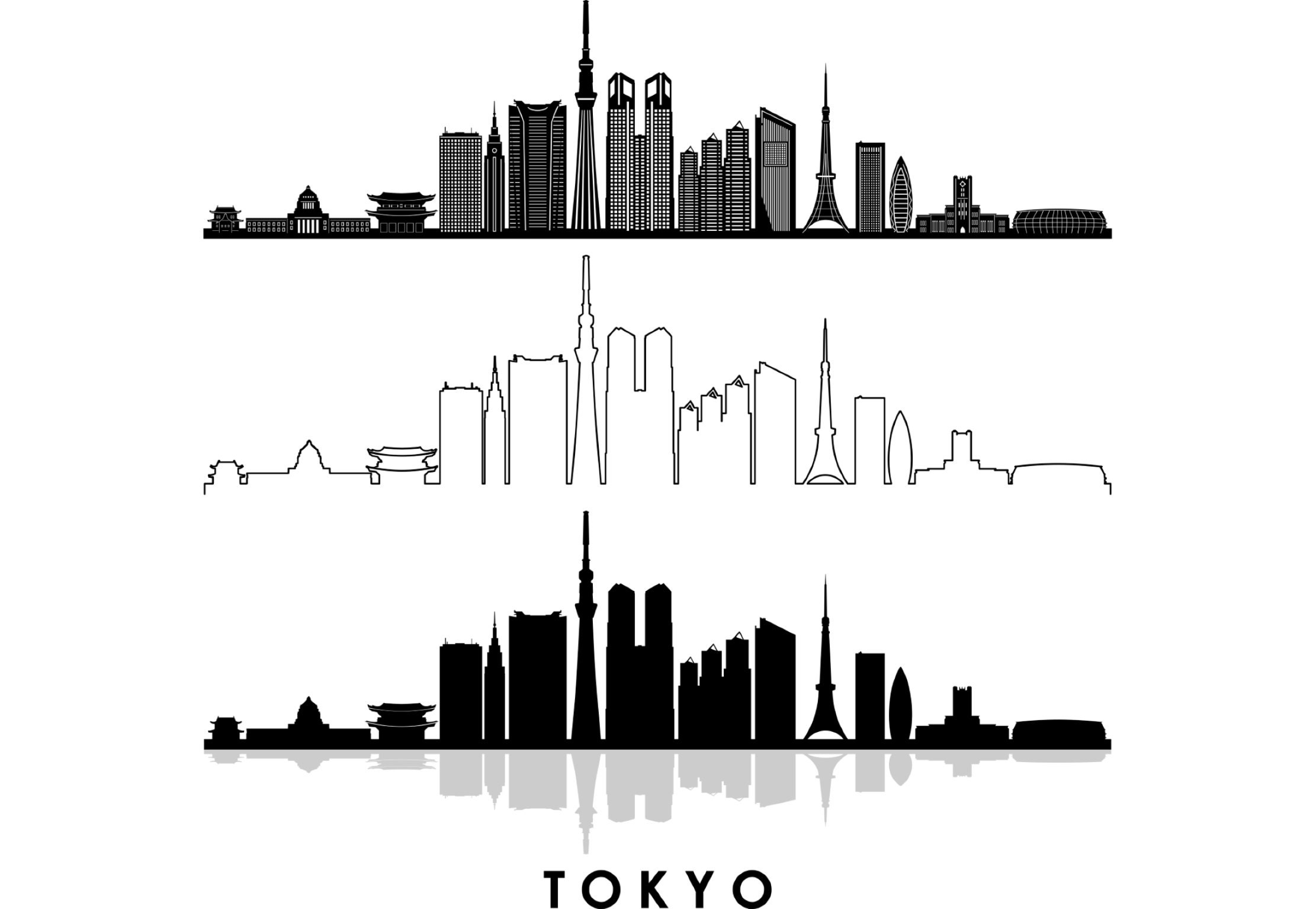The image depicts a stylized representation of the Tokyo skyline in three distinct formats, organized vertically from top to bottom. The top section features a detailed, grayscale rendering of Tokyo's buildings, which mix modern skyscrapers with traditional structures, including pagodas and a tower resembling the Eiffel Tower. The middle section presents a simplified version, showing only the black outlines of the buildings against a white background, devoid of any internal details or texture. The bottom section depicts an inverse silhouette, where the buildings are entirely black, contrasted against a white background. This section also includes a mirrored reflection of the black skyline in gray beneath it. At the very bottom of the image, the word "TOKYO" is prominently displayed in capital letters.